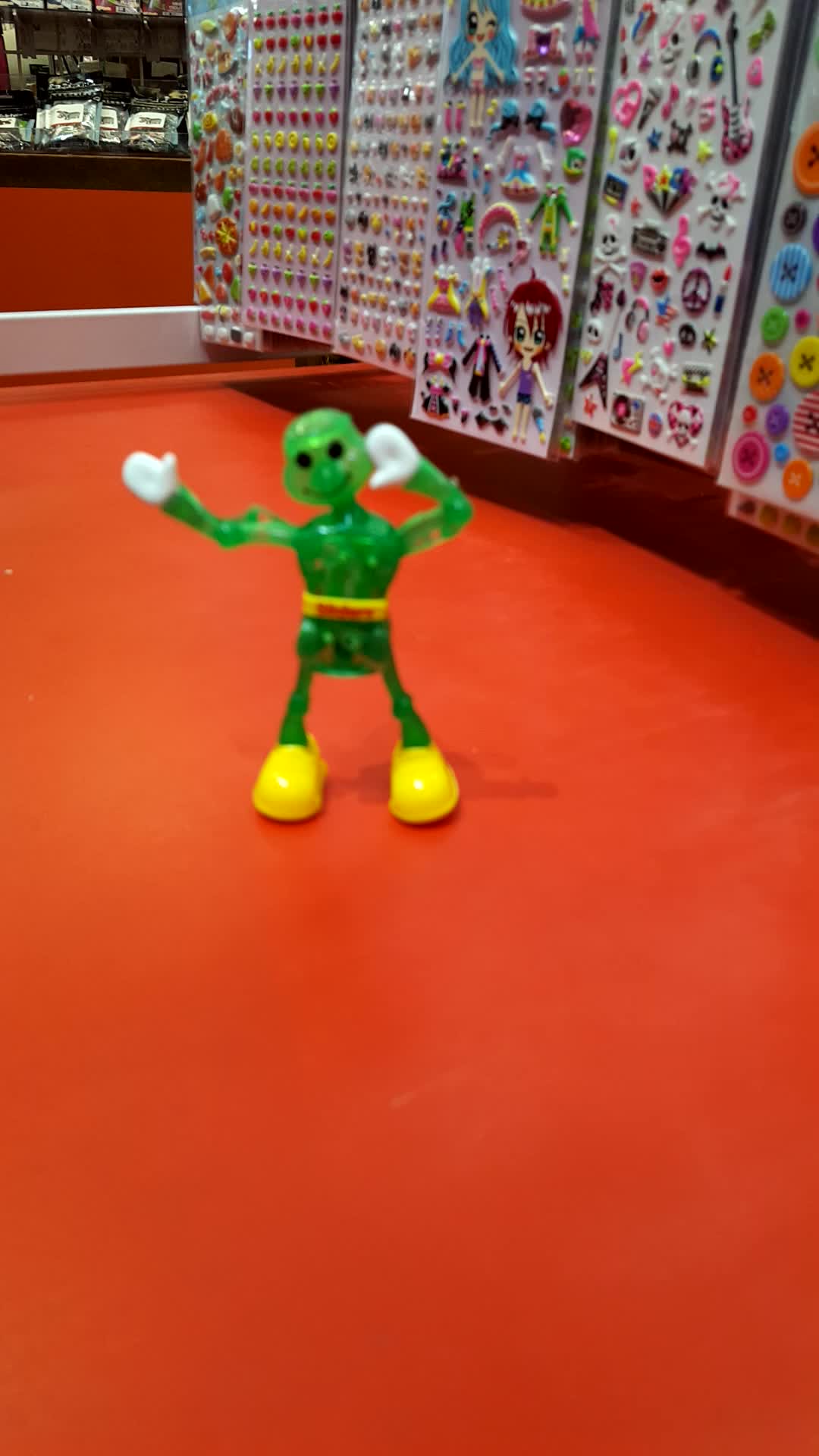In this detailed image, a small green action figure is positioned on what looks like the floor of a shop, characterized by an orange floor, a white trim, and an orange counter. The action figure is semi-transparent green, with white gloves, large yellow shoes, and a yellow belt adorned with red writing, although the text is somewhat blurry and illegible. Its face features black eyes and a black smile. This figure, with one arm extended upwards and the other bent at the elbow, stands just below and to the right of center in the image. The background includes a display of six rows of sticker packets hanging along the top third of the photograph, showcasing a variety of designs like hearts, characters, guitars, skulls, and buttons. This setting suggests that the photo was taken in a hobby store or an aisle filled with knickknacks, possibly targeting a younger demographic. The photo itself is a vertical rectangle, much taller than it is wide, accentuating the height of the store display compared to the small figure.